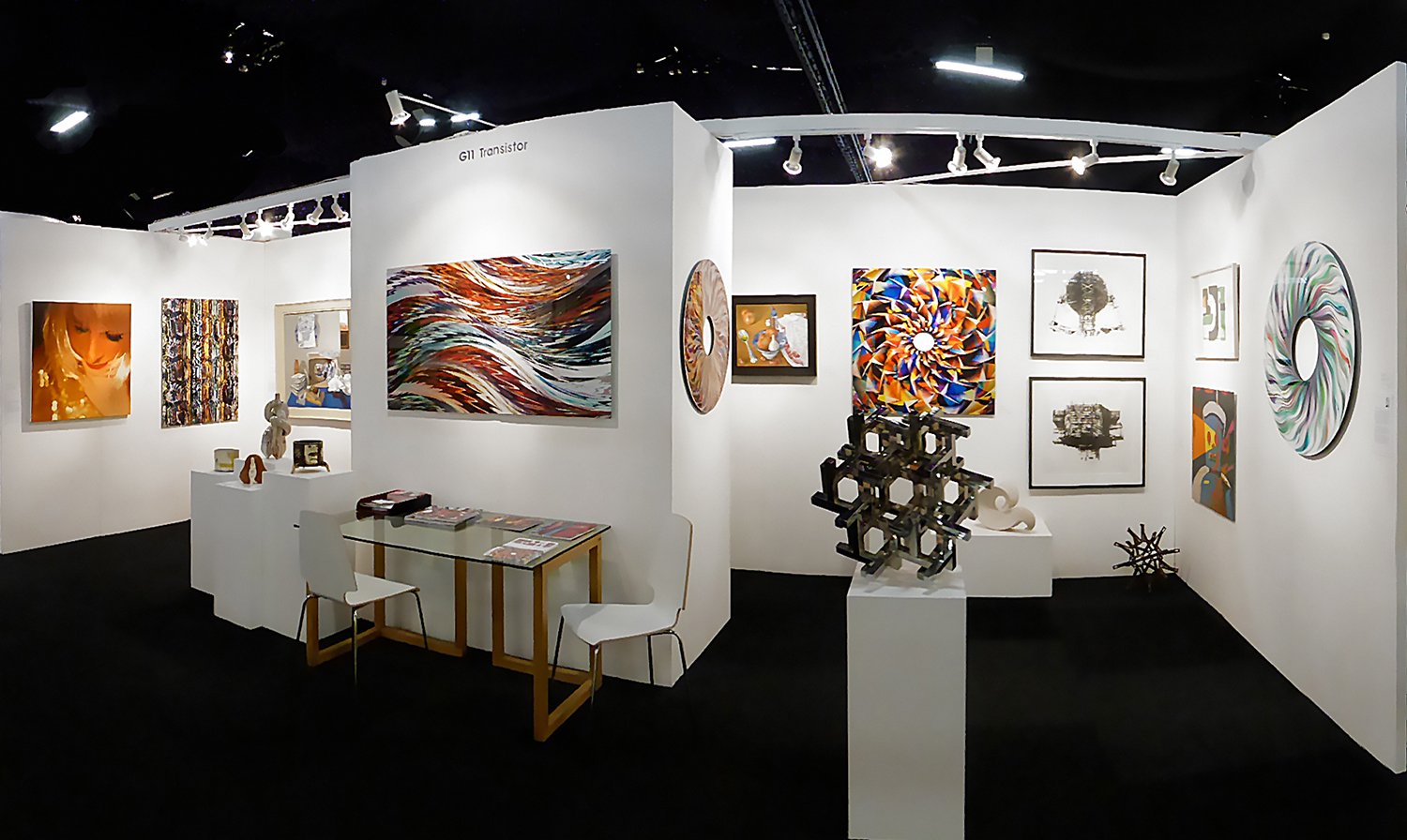The image depicts the interior of a meticulously arranged art gallery or museum, characterized by its stark white walls and black ceiling adorned with hanging lights. The gallery floor, covered in black carpet, accentuates the diverse collection of artwork displayed. 

Central to the scene is a prominent rectangular white structure with a clear glass table, wooden frame, and two chairs positioned in front of it, possibly serving as a security desk or receptionist area. The walls exhibit a variety of paintings, including a portrait of a veiled woman on the left and a vibrant modern art piece straight ahead to the right. Another striking artwork is a large circular piece on the far right, resembling a giant compact disc with red and light blue flares. 

In the middle of the room stands a tall white pedestal featuring a complex sculpture composed of dark brown angular forms and hexagonal patterns. Surrounding this central structure are additional paintings, including an abstract piece with flag-like strokes of red, white, and light blue. The gallery exudes a beautifully organized and thoughtfully curated display, likely showcasing the works of local artists.